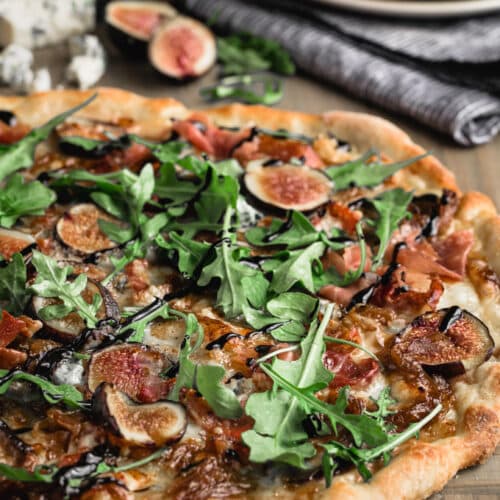This image captures a close-up of a gourmet, uncut pizza with a perfectly baked, hand-rolled golden brown crust. The pizza is lavishly topped with vibrant green arugula leaves, slices of figs showcasing a reddish interior with white rings, and roasted mushrooms. Crispy slices of pepperoni and possibly ham add a savory depth, while a zigzag drizzle of what appears to be a black balsamic reduction enhances its gourmet appeal. The cheese, although indistinct in type, displays a mouthwatering golden brown melt. The pizza rests on what seems to be a brown wooden table, and in the background, slightly out of focus, is a gray rolled-up tablecloth and a plate on the top right. The top left reveals white designs, potentially an out-of-focus glass, and another vegetable item with a red interior. This meticulously detailed setting underscores the artisanal quality and intricate presentation of the pizza.